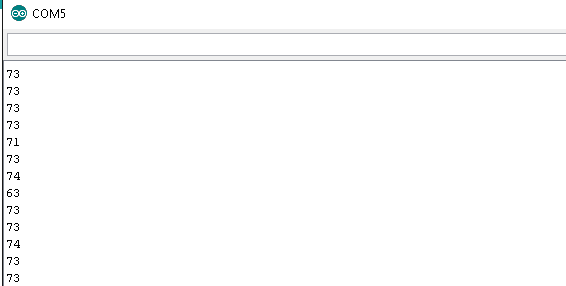The image displays a distinctive logo within a small green circle, featuring two smaller white circles positioned closely together, reminiscent of eyeglasses. Beneath the green circle, in bold, black, uppercase letters, it reads "COM5," though it could also be interpreted as "C0M5" due to the typography. Adjacent to the logo, there appears to be a search bar, outlined in gray, resembling a large rectangle.

Below this, a series of numbers are neatly listed in a single line: 73, 73, 73, 73, 71, 73, 74, 63, 73, 73, 74, 73, 73. This line arrangement is akin to an Excel spreadsheet but lacks grid lines, providing an organized yet simplified appearance. There is a single black line at the very beginning of the number sequence, resembling the start of a row.

The only vivid color in the image comes from the green circle logo. Additionally, in the upper left-hand corner, there is a very small green rectangle which might go unnoticed without good eyesight. This combination of elements gives the impression of a well-structured yet minimalist design.